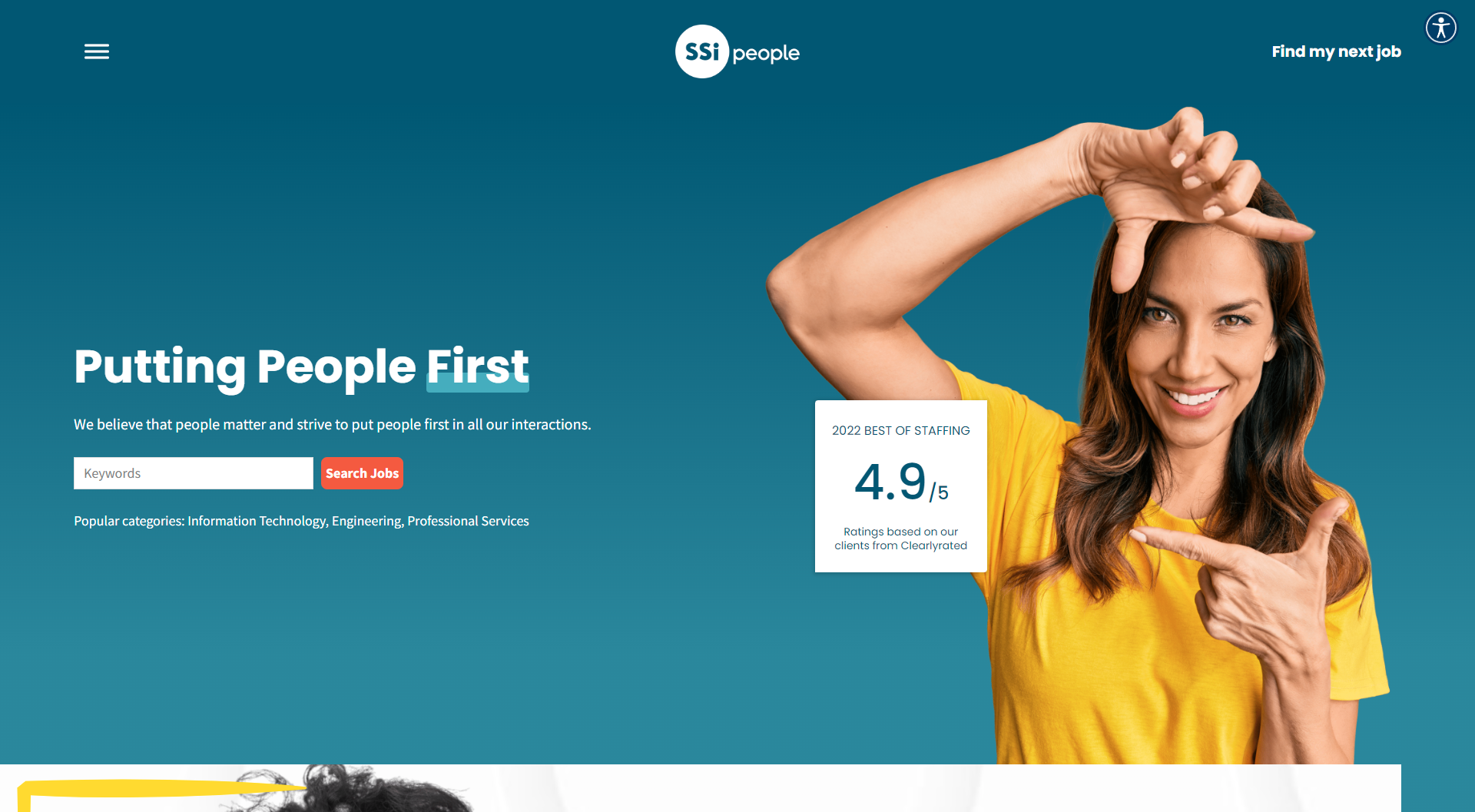This is a detailed screenshot of the SSI People website. At the top center, "SSI People" is prominently displayed, with "SSI" encased in a white circle. On the far left side, there are three horizontal bars representing a menu icon. 

The top right corner features the options "Find My Job" and "My Next Job," accompanied by a stick figure icon inside a blue circle. The entire page has a blue background.

On the right side of the image, a woman with long brown hair extending past her shoulders is wearing a yellow short-sleeve shirt. She is smiling and making a gesture with her hands as if framing a photograph. Next to her, there's a white box that reads, "2022 Best of Staffing 4.9 out of 5 stars ratings based on our clients from ClearlyRated."

On the left side of the page, large white text declares, "Putting People First." Underneath, in a smaller font, it reads, "We believe that people matter and strive to put people first in all of our interactions." 

At the bottom, there is a prominent red button labeled "Search Jobs," accompanied by a white rectangular box for typing in keywords. Below this search box, it lists popular categories: Information Technology, Engineering, and Professional Services.